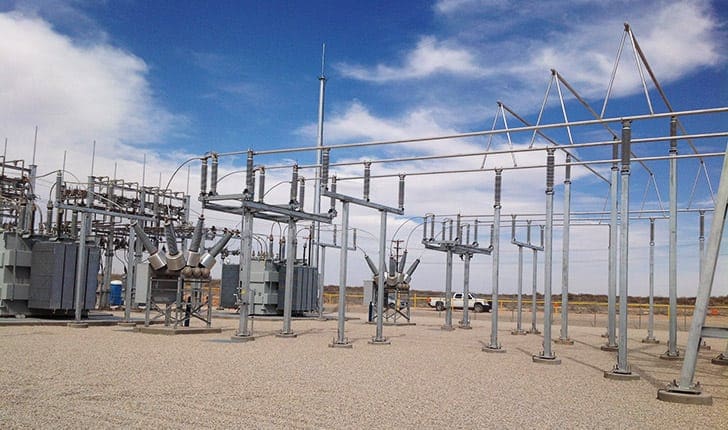The image depicts an outdoor power substation situated on a light gray and beige gravel plot. The foreground prominently features a variety of tall, metallic electrical equipment with an array of vertical and horizontal poles, transformers, and piping. These components, mostly in dull silver, stretch across the middle section of the photo, giving a robust, industrial appearance. On the left, in the background, sit large rectangular metal containers topped with more poles. The backdrop of the scene shows a bright blue sky accented by feathery white clouds, indicating a clear day. Towards the center of the image, behind the equipment, a white pickup truck is parked along a yellow fenced area, possibly belonging to maintenance service technicians. Additionally, a small blue and white outhouse can be seen on the left side, partially obscured by the array of equipment. The color palette of the photo includes blue, white, gray, silver, tan, and hints of brown and red, contributing to the detailed industrial atmosphere of the substation.